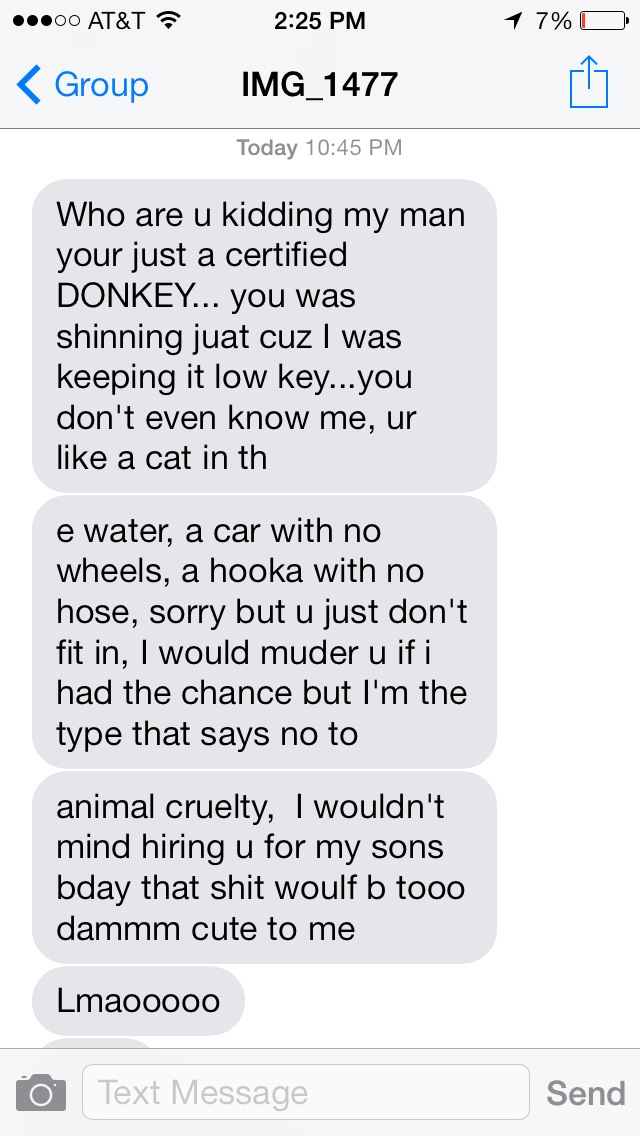The image is a screenshot of a text message conversation on a cell phone, captured at 2:25 PM with a 7% battery level, depicted by a symbol in the upper right corner. The title at the top reads "IMG_1477" and the carrier is AT&T. The message thread starts with "today 10:45 PM," and the text message in grey bubbles from one person reads: "Who are you kidding? My man, you're just a certified donkey. You were shining just because I was keeping it low key. You don't even know me. You're like a cat in the water, a car with no wheels, a hookah with no hose. Sorry, but you just don't fit in. I would murder you if I had the chance, but I'm the type that says no to animal cruelty. I wouldn't mind hiring you for my son's B-day. That shit would be too damn cute to me. L-M-A-O." The screenshot also shows a partial text input bubble at the bottom.